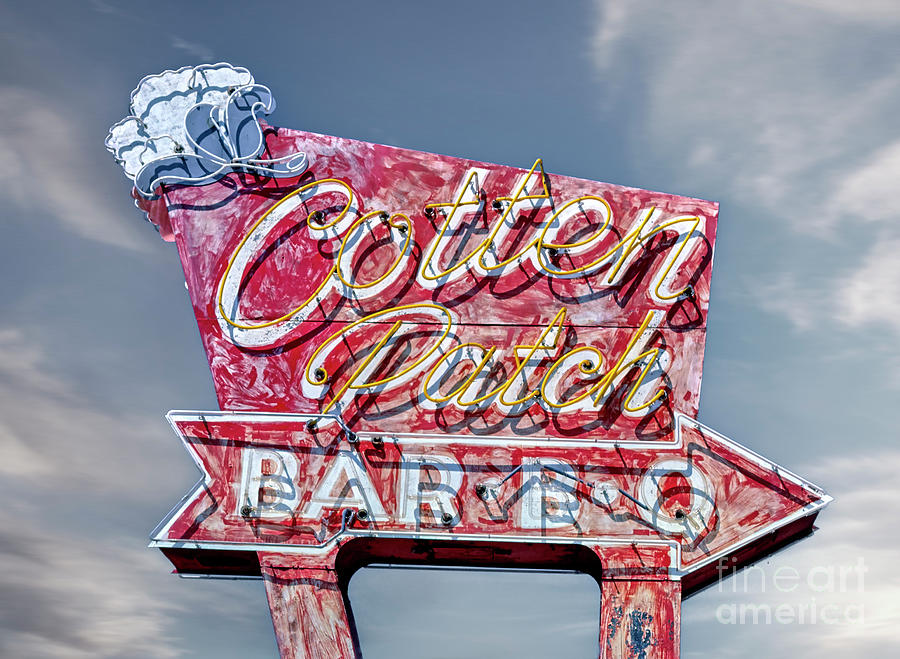Against a backdrop of a grayish-blue sky dotted with sparse, wispy white clouds, stands a weathered, towering sign. Once vibrant with neon lights, the sign has now faded to a deep, washed-out red. At the top left corner of the sign, there's a depiction of a cotton flower.

Dominating the sign are the words "Cotton Patch," spelled out in large, cursive letters. "Cotton" and "Patch" are prominently displayed with a mix of yellow and white accents that hint at their former brilliance. Below the main heading is a distinct red arrow, outlined in white, pointing to the right. Within the arrow are the words "BAR B.Q.," capitalized in white letters.

On the right lower edge of the image, almost blending with the clouds, the watermark "Fine Art America" appears faintly in red, hinting at the image's artistic provenance.